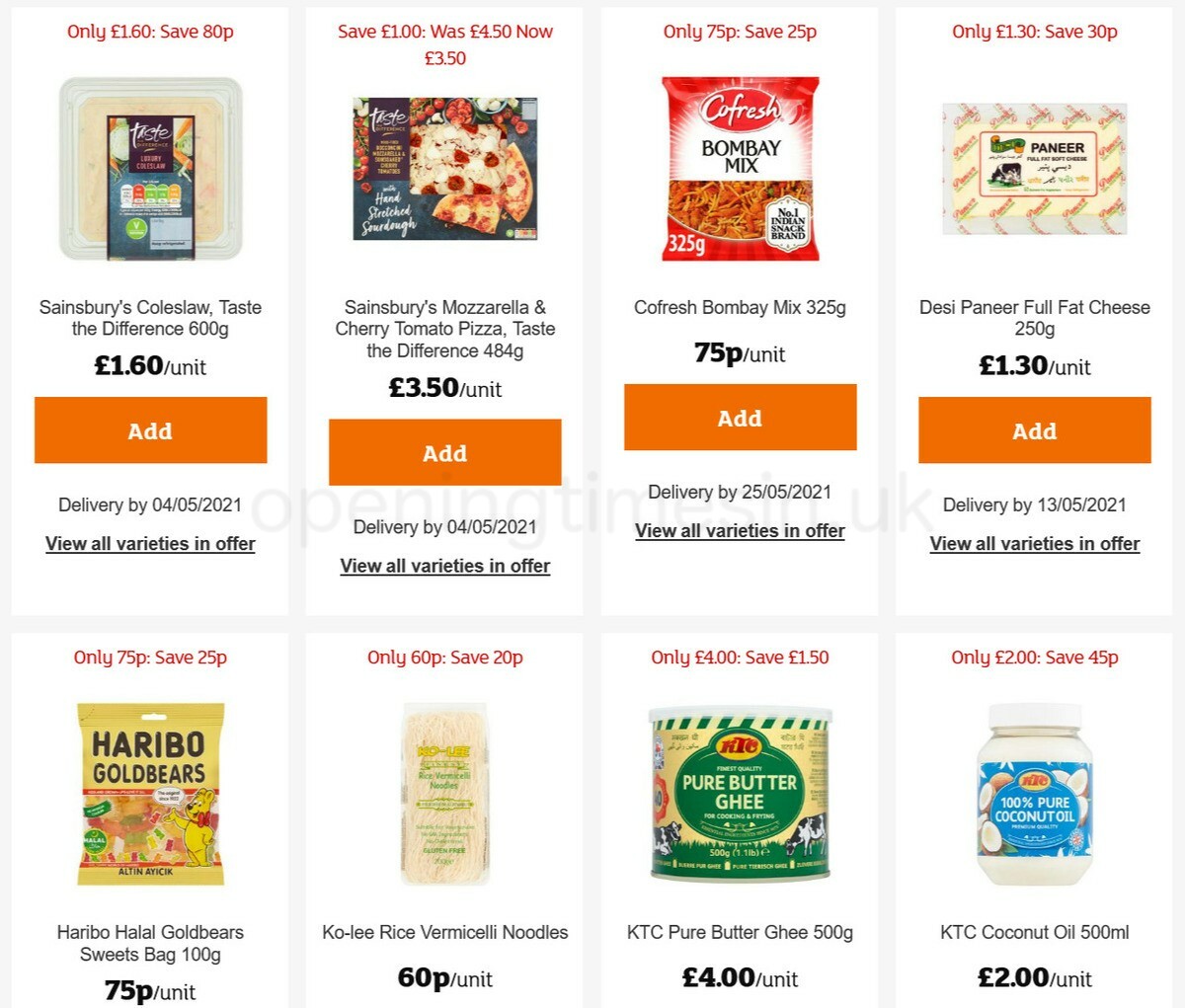This screenshot showcases a diverse selection of food products available for purchase from an online store. The page displays eight different items, each detailed with price, size, and some additional information.

Starting from the top left:

1. **Sainsbury's Coleslaw** – This is a "Taste the Difference" product weighing 600 grams, priced at £1.60 per unit. An orange "Add" button is provided, and the delivery date is noted as 04-05-2021. There is also a link to "View all varieties in offer."

2. **Haribo Halal Gold Bears** – This product is a 100-gram bag of Haribo gold bear sweets, priced at 75 pence per unit.

Moving to the top center:

3. **Sainsbury's Mozzarella Cherry Tomato Pizza** – Another "Taste the Difference" product, this pizza comes in a boxed package with an image of the pizza on it. It is priced at £3.50 per unit and shares the same add button, delivery date, and variety link details as the coleslaw.

4. **Coli Rice Vermicelli Noodles** – Displayed with a picture of a bag of white noodles, this product costs 600 pence per unit.

Shifting toward the top right:

5. **Cold Fresh Bombay Mix** – This item appears in a chip-style bag and is priced at 75 pence per unit, accompanied by the same add, delivery, and variety buttons as earlier items.

6. **KTC Pure Butter Ghee** – This ghee comes in a 500-gram container, priced at £4 per unit, with a note indicating a savings of £1.50 per unit.

In the bottom row, from left to right:

7. **Desi Paneer Full Fat Cheese** – Weighing 250 grams and priced at £1.30 per unit (with a saving of 30 pence), this cheese features the same set of interactive buttons.

8. **KTC Coconut Oil** – This product is presented in a 500-milliliter jar with a visible label, priced at £2 per unit.

Each product is neatly outlined with a photo and concise details, making it easy for users to browse and make selections based on their preferences.